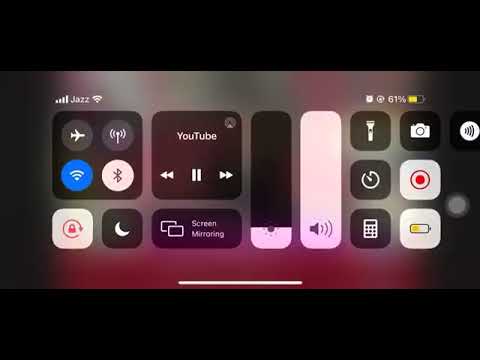The image is a wide rectangular screenshot from an iPhone, which appears to be in portrait mode, as indicated by the black bars on the top and bottom cropping the view. The screenshot depicts the iPhone's Control Center, which is accessed by swiping down from the top of the screen. The background is blurry and displays patches of gray, red, and green colors, adding to the layered appearance of the interface.

In the top left corner, the signal strength is depicted by four ascending bars, next to the network name "jazz" and a Wi-Fi signal icon. The Control Center itself is composed of several transparent black squares with curved edges, each containing a variety of toggle switches and shortcuts.

Key elements featured in this menu include icons for Airplane Mode, Wi-Fi, Bluetooth, Night Mode (depicted by a moon icon), and Screen Mirroring. There's also a section to control a YouTube video with play, pause, fast forward, and rewind buttons. Additional controls include volume and brightness sliders; the volume indicator is white, while the brightness bar sits low with a majority of the bar remaining black. Other icons in the Control Center include toggles for screen recording (indicated by a red circle), the camera, flashlight, calculator, timer, as well as an icon for accessing Spotify.

In the top right corner, there is a battery icon showing a 61% charge with a yellow fill, signifying a partially full battery. A small clock icon sits beside the battery indicator. At the bottom of the screenshot is the white gesture bar typical of an iPhone. This detailed view highlights the extensive range of functionalities accessible directly from the iPhone's Control Center.